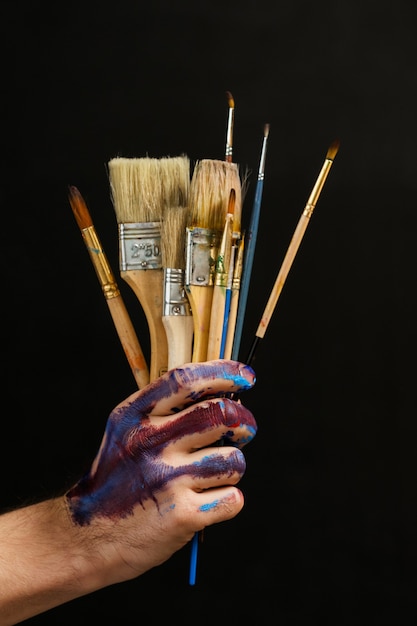The photograph features a right hand covered in mostly purple and a bit of blue paint, more concentrated on the index, middle, and ring fingers, with lesser amounts on the pinky. The hand grips a collection of art paintbrushes of various sizes and colors. Prominently, there are two larger, thicker brushes at the center surrounded by smaller, fine-tipped brushes, all with different colored handles. The background is entirely black, which highlights the vivid colors of the paint and the assortment of the well-used brushes.